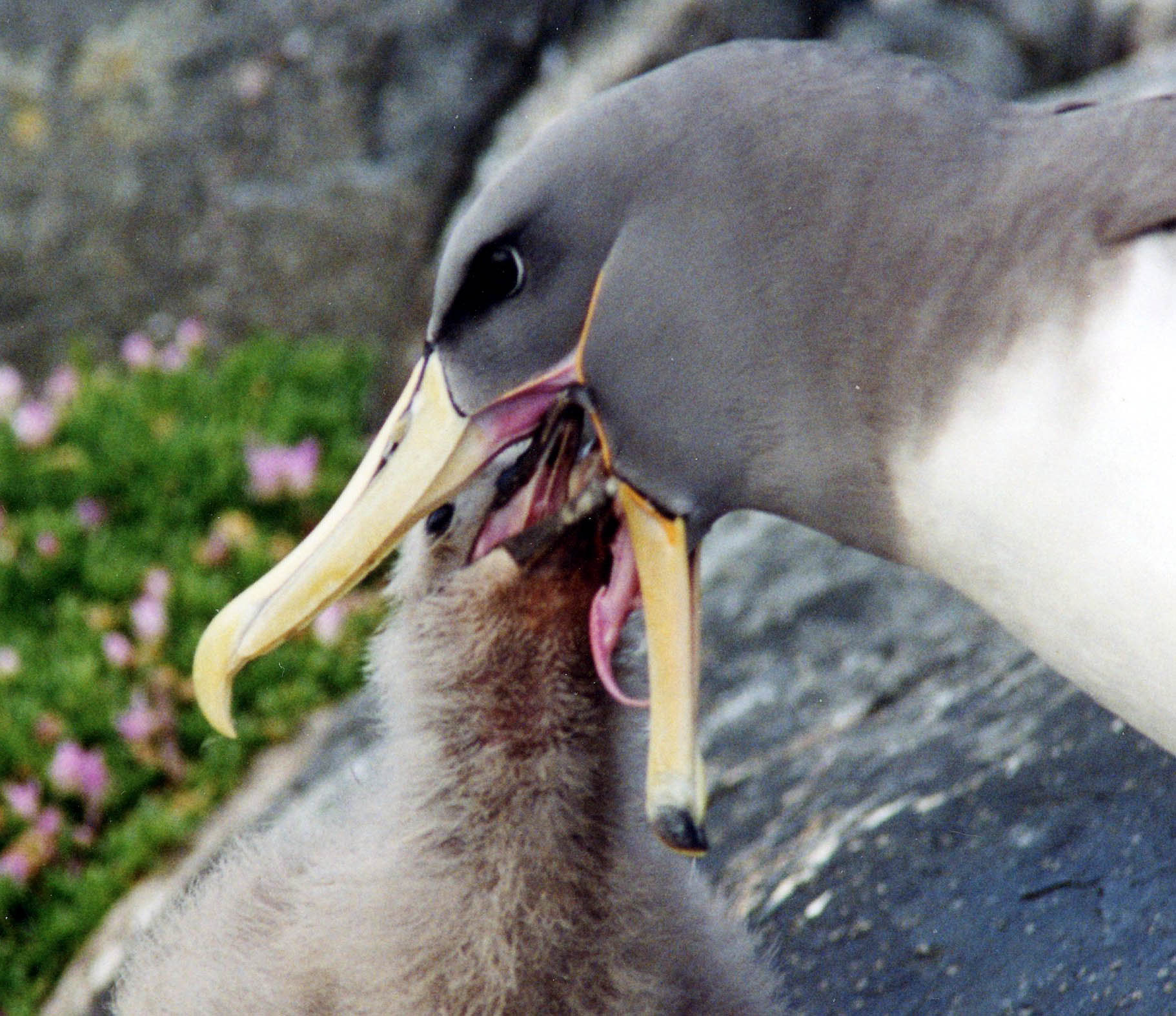In this close-up image, an adult penguin with a gray head and yellow beak is intricately feeding a baby penguin. The adult is bending down, with its mouth wide open, as the baby's beak reaches deep into the adult's mouth, almost down its throat, to consume the regurgitated food. The adult penguin's striking features include its black eyes and a white chest contrasted by black wings. The baby penguin is predominantly tan with a distinctive black streak down its chest and has a black beak. Both penguins are perched on a rock, with a backdrop that includes some green foliage and pink flowers, adding a touch of natural beauty to the scene. The closeness of the shot highlights the tender interaction, capturing only the head and a snippet of the neck of the adult penguin and the fluffy, brown-and-white coloration of the baby.